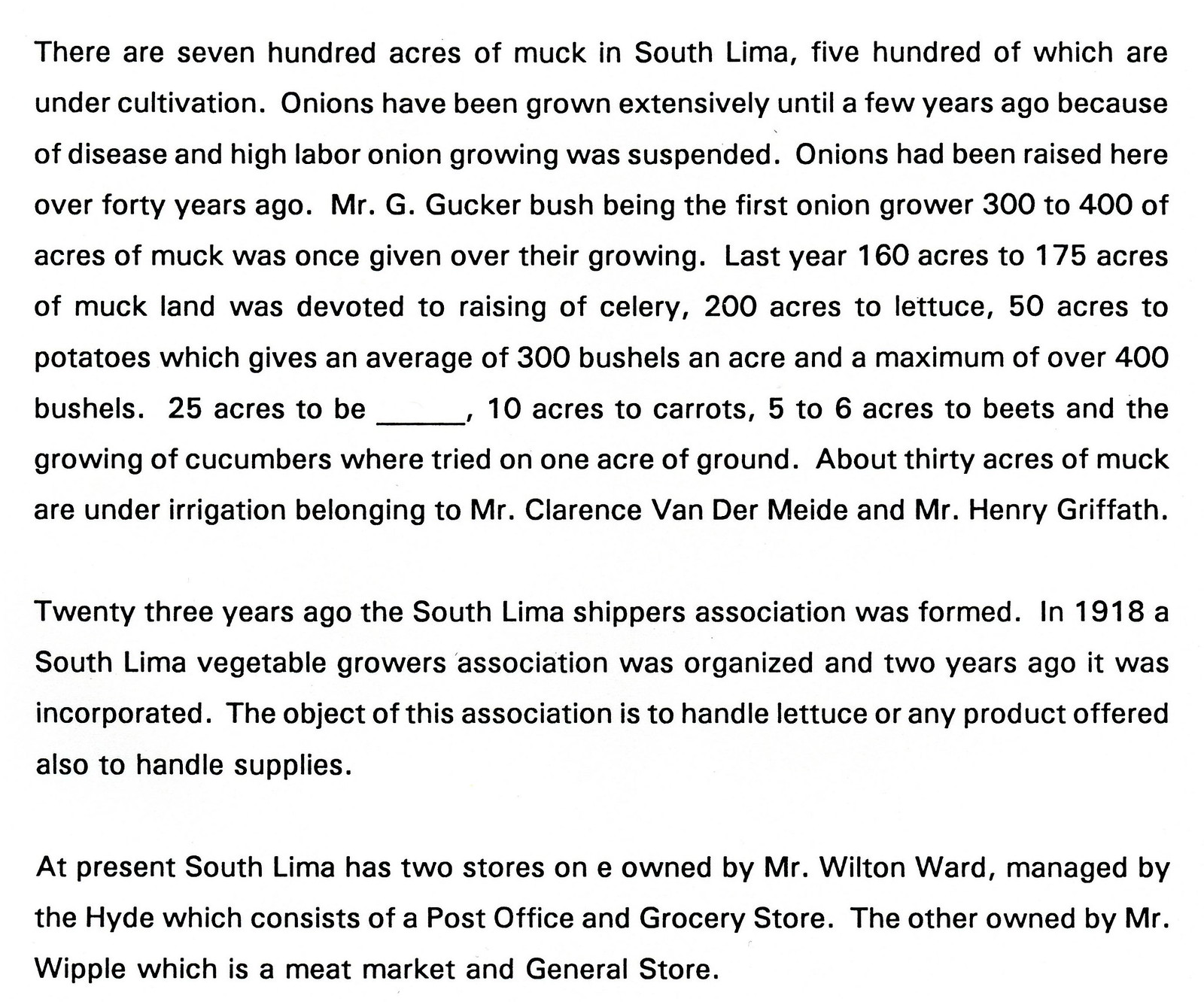The image consists of black text set against a white background, taking the form of three paragraphs without indentation and double spacing between them. The top half of the image is occupied by the first and largest paragraph, which begins with: "There are 700 acres of muck in South Lima, 500 of which are under cultivation." It details the history and current use of the land, mentioning that onions were extensively grown until a few years ago when disease and high labor led to the suspension of onion growing. Onions had been grown for over 40 years, with Mr. G. Gucker Bush being the first to cultivate them. 300 to 400 acres were once dedicated to onions. Last year, 160 to 175 acres were used to raise celery, 200 acres for lettuce, 50 acres for potatoes (yielding an average of 300 bushels per acre and a maximum of over 400 bushels), 25 acres for an unspecified crop, 10 acres for carrots, 5 to 6 acres for beets, and one acre for cucumbers. About 30 acres are under irrigation by Mr. Clarence Vandermyde and Mr. Henry Griffith.

The second paragraph states: "23 years ago the South Lima Shippers Association was formed." It further adds that the South Lima Vegetable Growers Association was organized in 1918 and incorporated two years ago to handle lettuce and other products as well as supplies.

The bottom paragraph mentions that currently, South Lima has two stores on E Street. One is owned by Mr. Wilton Ward and managed by the Hyde, housing a post office and grocery store. The other store, a meat market and general store, is owned by Mr. Whipple.